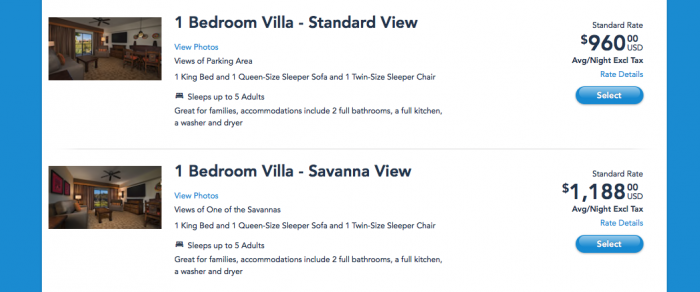This image is a screenshot of the booking section from a hotel's website. Displayed are two accommodation options, each depicting detailed offerings and pricing.

1. The first option is for a "One-Bedroom Villa with Standard View." A small thumbnail image suggests this is the living room area of the villa. This choice includes a view of the parking area. The villa comfortably sleeps up to five adults, thanks to one king bed, one queen-sized sleeper sofa, and one twin-sized sleeper chair. Designed with families in mind, it includes two full bathrooms, a full kitchen, and a washer and dryer. The standard rate for this option is $960 USD per night, excluding taxes. Buttons to “View Photos," "See Rate Details," and "Select This" are available.

2. The second option is a "One-Bedroom Villa with Savannah View." Again, a small thumbnail image hints at the appealing living room space. Guests can expect views of one of the savannahs. This villa also accommodates up to five adults with one king bed, one queen-sized sleeper sofa, and one twin-sized sleeper chair. Like the standard view villa, it includes two full bathrooms, a full kitchen, and a washer and dryer. The standard rate here is higher, at $1,188 USD per night, excluding taxes. Similarly, it has buttons for “View Photos," "See Rate Details," and "Select This."

Both options emphasize family-friendly accommodations with modern conveniences and beautiful views.